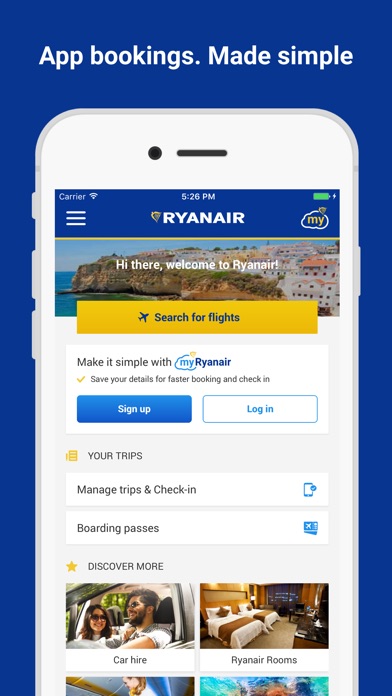**Descriptive Caption:**

On a serene blue background, the header prominently displays the phrase "App Bookings Made Simple" in white text. Below this, a smartphone illustration is central to the design. 

At the top of the phone screen, two small black icons—a circle and a dash—are visible. The status bar features a blue rectangle labeled "carrier," accompanied by a Wi-Fi symbol. Although the exact time is unclear, a green battery indicator is situated on the right.

Under the status bar, there's a section with three horizontal lines forming a symbol that’s too small to decipher, followed by the text "RYANAIR." 

A cloud-shaped graphic containing the word "my" in yellow appears next to the aforementioned elements. Below this, a scenic illustration showcases a city by the water along with a welcoming message: "Hi there, welcome to Ryanair." 

Prominently positioned is a yellow rectangle with an airplane icon next to the text "Search for flights." Adjacent to it is a white rectangle that reads, "Make it simple with my Ryanair," framed by a cloud graphic and adorned with a small yellow dot. The word "my" is in light blue and "Ryanair" in dark blue. 

Further down, a yellow checkmark is followed by the text "Save your details for faster booking and check-in." Below that are two buttons: a blue rectangle labeled "Sign up" and a blue-outlined rectangle for "Log in."  

Continuing down the interface, a yellow and orange rectangle labeled "Your trips," sits above a white rectangle that states, "Manage trips and check-in." Adjacent to this, an image of a phone with a dot on the right-hand side is shown, and another white rectangle labeled "Boarding passes."

On the lower part of the screen, there is an indistinct blue image and a star icon with the text "Discover more." Additional visuals depict options for “Car hire,” “Ryanair rooms,” and parts of two pictures beneath these options. The overall design is clean, user-friendly, and encourages seamless interaction for booking flights and managing travel details through the Ryanair app.